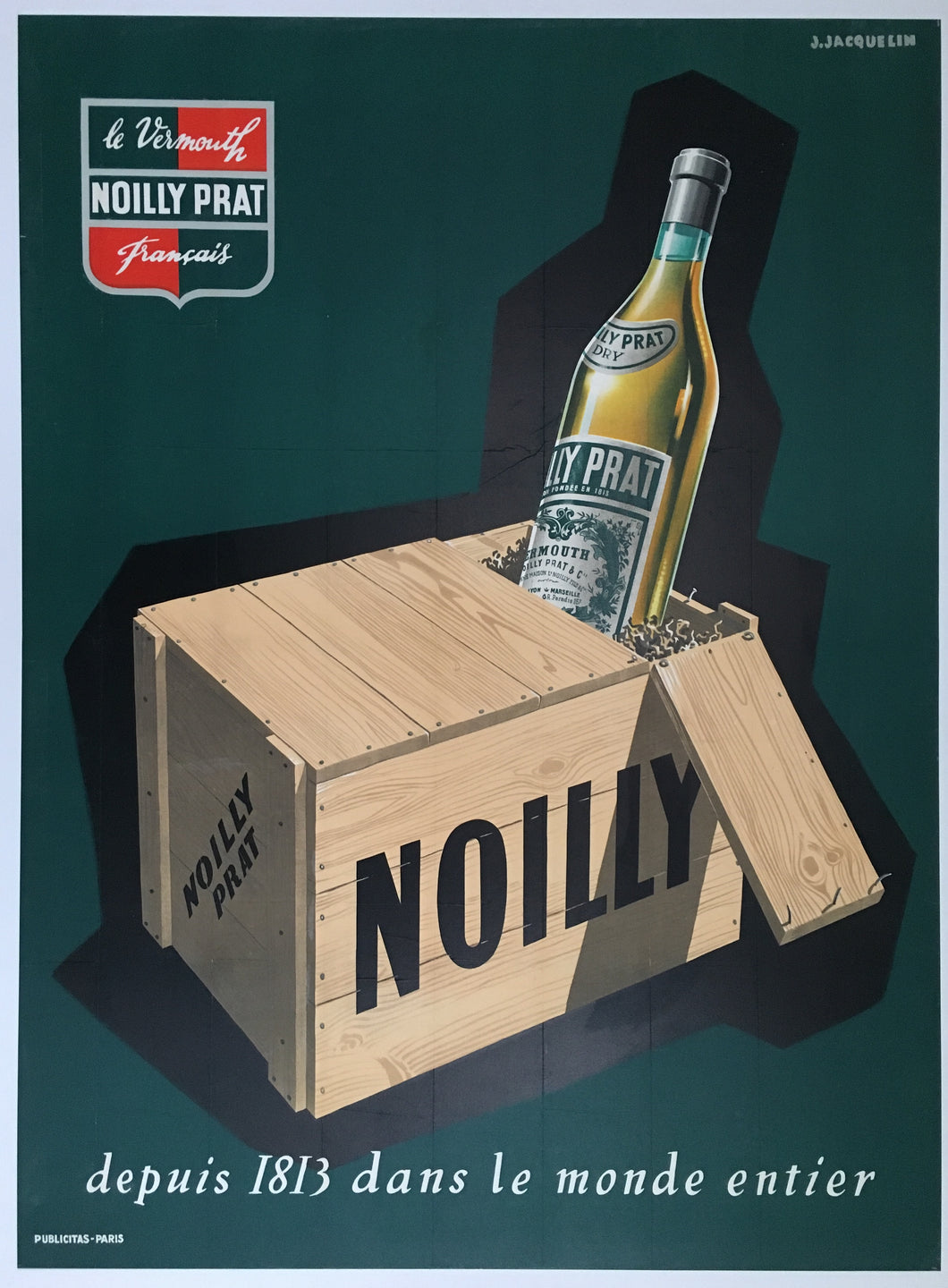This image is a vintage-styled, illustrated advertisement for Noilly Prat Vermouth, predominantly in French, reminiscent of a cartoon drawing. The focal point is a prominent olive green bottle of vermouth with a silver and darker green label, emerging from an open brown wooden crate marked "NOILLY PRAT" in bold capital letters on both the front and left sides. The dark green background enhances the imagery, casting a black shadow from the box and bottle, giving depth and emphasizing the product. In the top left corner, there is a logo resembling a shield or banner flag, colored in dark green and red, inscribed with "VERMOUTH NOILLY PRAT FRANCAISE." The bottom text of the image reads: "DEPUIS 1813 DANS LE MONDE ENTIER," indicating the brand's establishment in 1813. Additionally, the corner of the image bears the inscription "Publicitas Paris," likely attributing to the advertising agency. No human figures are present in the image, maintaining the focus on the advertised vermouth.